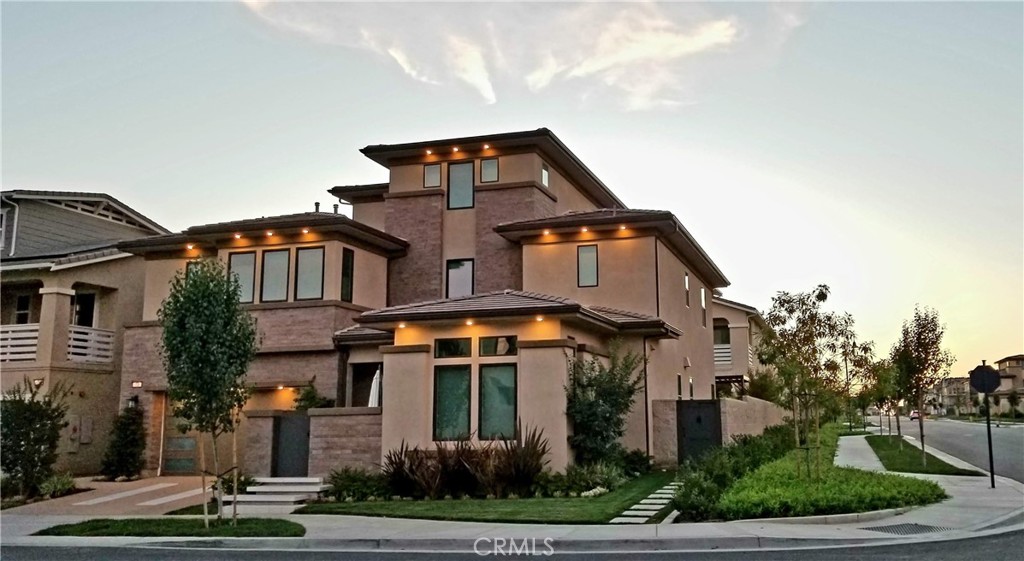This color photograph, taken at sunset, captures a modern, light brown house situated on the corner of a suburban street. The sky occupies half the image, showcasing a halo and cloud formations that beautifully frame the structure. The house features a unique split-level design with four distinct sections: the ground level with a square front, two two-story segments on either side, and a tall, cube-like third story in the center back. The facade is accented by numerous rectangular windows. In the foreground, a sidewalk with a rounded edge curves around the house, flanked by small patches of green grass, a few small bushes, and a little tree. The letters "CRMLS" appear at the bottom of the photograph, near where the curb meets the street.